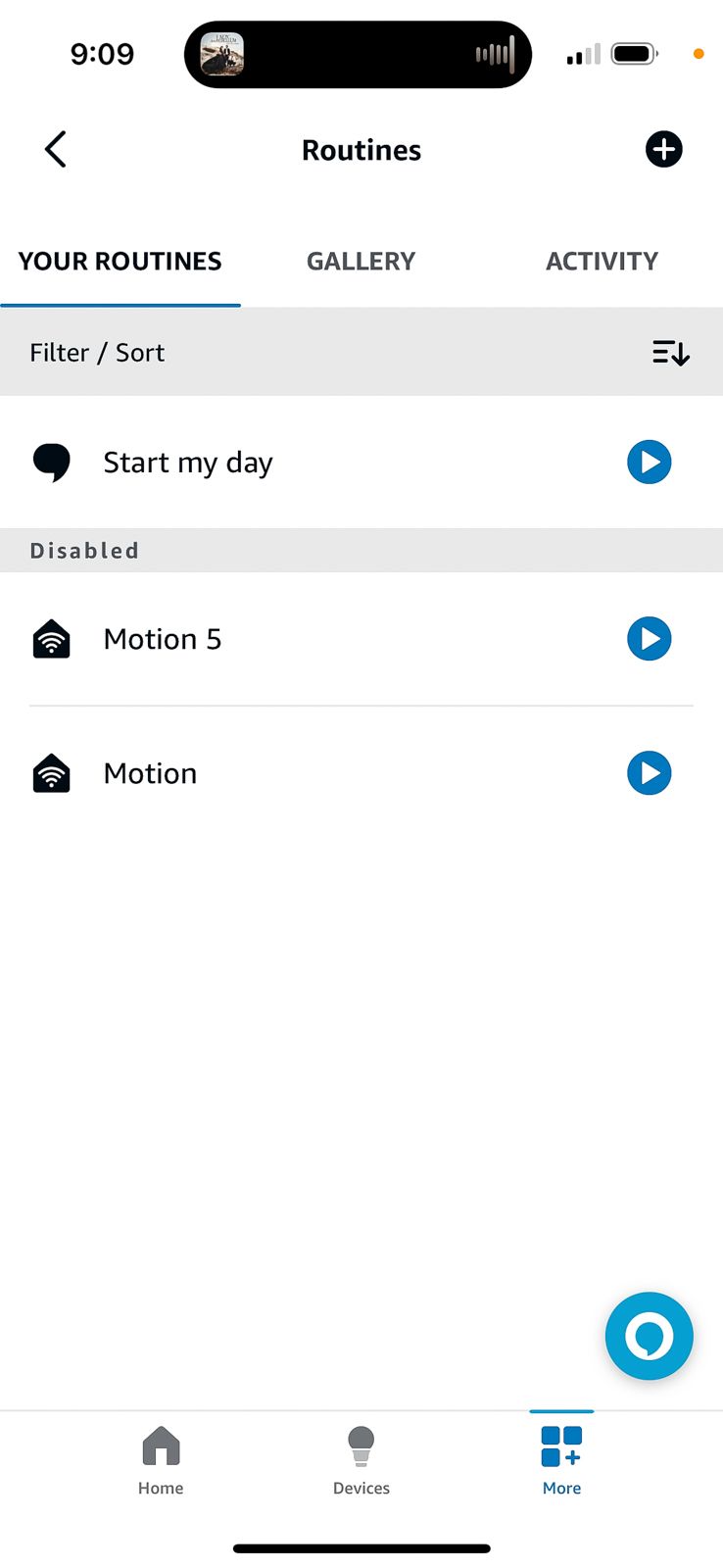This image is a screenshot from a mobile Amazon device, possibly illustrating a section of the Alexa app. The screen has a white background, resembling a menu interface. At the top, standard icons for battery life and cellular signal are visible, similar to those on a smartphone. However, an unmistakable element is the blue Alexa logo situated in the bottom right corner, suggesting the app is being used.

Heading the screen is the title "Routines" in bold black text, aligned with a plus icon that likely allows users to add new routines. The interface is divided into three clickable tabs at the top: "Your Routines," "Gallery," and "Activity." The "Your Routines" tab is currently selected.

Displayed under the selected tab are various routines created by the user. The first routine listed is named "Start My Day," accompanied by a speech bubble icon, indicating it might involve voice commands or notifications. Below this, in a section labeled for disabled routines, are two routines illustrated with house icons incorporating Wi-Fi signals, named "Motion 5" and "Motion."